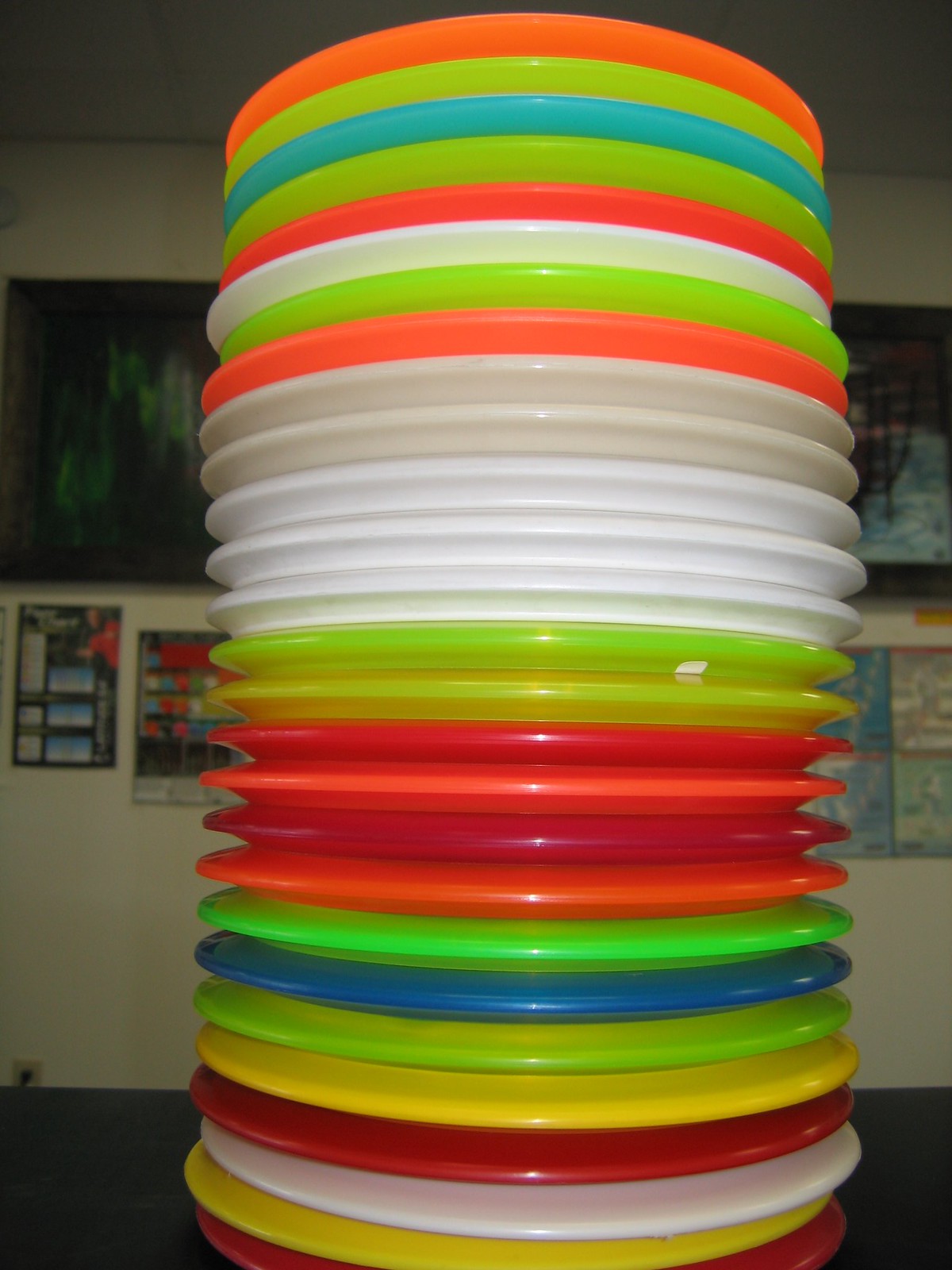The image displays a high stack of neon-colored plastic plates on a dark-colored table. The plates come in various bright hues including neon red, neon green, white, beige, neon orange, and neon yellow. The background features a beige wall adorned with multiple paintings. Two larger paintings, predominantly dark green with white accents, are accompanied by smaller ones below. One of the paintings appears to depict a map. Notably, an optical illusion makes it seem as though the orange plate at the top of the stack almost meets the ceiling; however, it does not. Additionally, one painting on the right features an animal by a river. The plates, although described by one voice as glass and ceramic in differing hues, are consistently shared as colorful and varied in shape and material, emphasizing a vibrant and eclectic collection against a simple and serene backdrop.